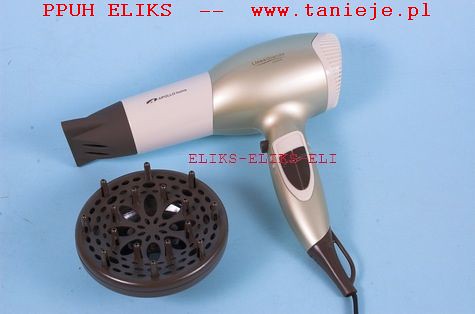This detailed photograph showcases a hair dryer with a predominantly silver body accented by white in the middle and black elements including the end, cord, and buttons. The hair dryer is lying on a light blue background, accompanied by its black attachments—a spiky diffuser for frizzier, curlier hair, and a thinner nozzle aimed at straightening hair. Above the hair dryer, red text reads "P-P-U-H-E-L-I-K-S-DASH-DASH-W-W-W-DOT-T-A-N-I-E-J-E-DOT-P-L," while smaller red text in the center spells "E-L-I-K-S-DASH-E-L-I-K-S-DASH-E-L-I." Additionally, the observed words suggest the presence of a website, further highlighted by the "www" prefix and dots between segments, indicating it's in a non-English language.